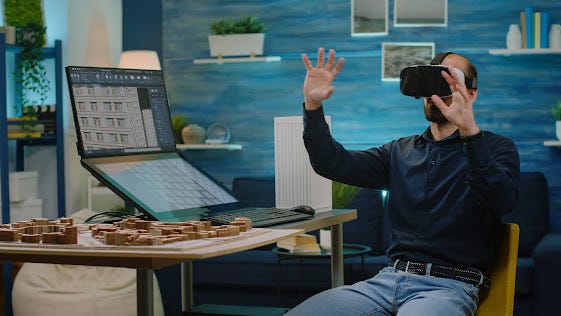In this photograph, a man is sitting in a yellow chair in what appears to be a living room or study. He is wearing a dark navy, long-sleeve pullover with buttons down the front, light-colored blue jeans, and a black belt. A VR headset with straps over the top and around the sides of his head covers his eyes, and he has his right and left hands raised, seemingly interacting with a virtual environment. To his left is a table holding an open laptop and various wooden pieces or tools. The background features a blue wall adorned with three pictures, shelves holding a plant and some books supported by two vases used as bookends. Behind him, a dark blue couch is also visible.